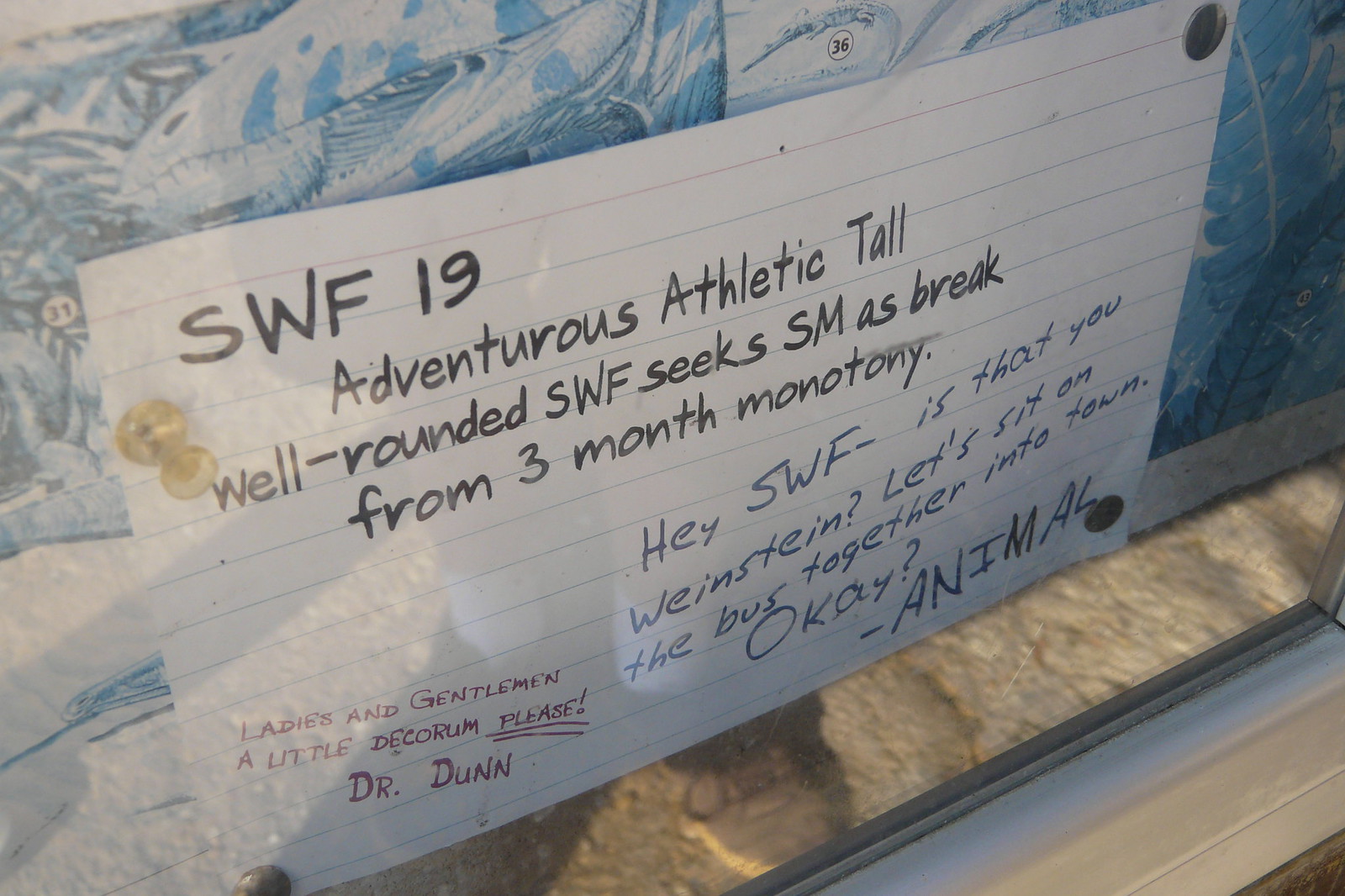The image depicts a white 3x5 note card tacked to a floral-patterned wall in shades of blue and white, possibly next to a window or a mirror. The note card is secured by four pins: a plastic pin on the upper left and flat, round metal pins on the other three corners. The background of the wall includes what appears to be a dinosaur's mouth and some kind of fauna in blue tones.

The note card features bold black marker text that reads: "SWF-19 Adventurous, Athletic, Tall. Well-rounded, SWF seeks SM as a break from three-month monotony." The majority of the image is dominated by this text.

In the bottom left corner of the card, written in dark red ink, it says: "Ladies and gentlemen, a little decorum please, Dr. Dunn."

In the bottom right corner, written in blue ink, there is a message that reads: "Hey SWF, is that you Weinstein? Let's sit on the bus together into town, okay? Animal."

Additionally, part of a window frame with black, blue, and lighter gray strips is visible at the bottom of the image, and the surface beneath the card appears to be a light brown wooden color.